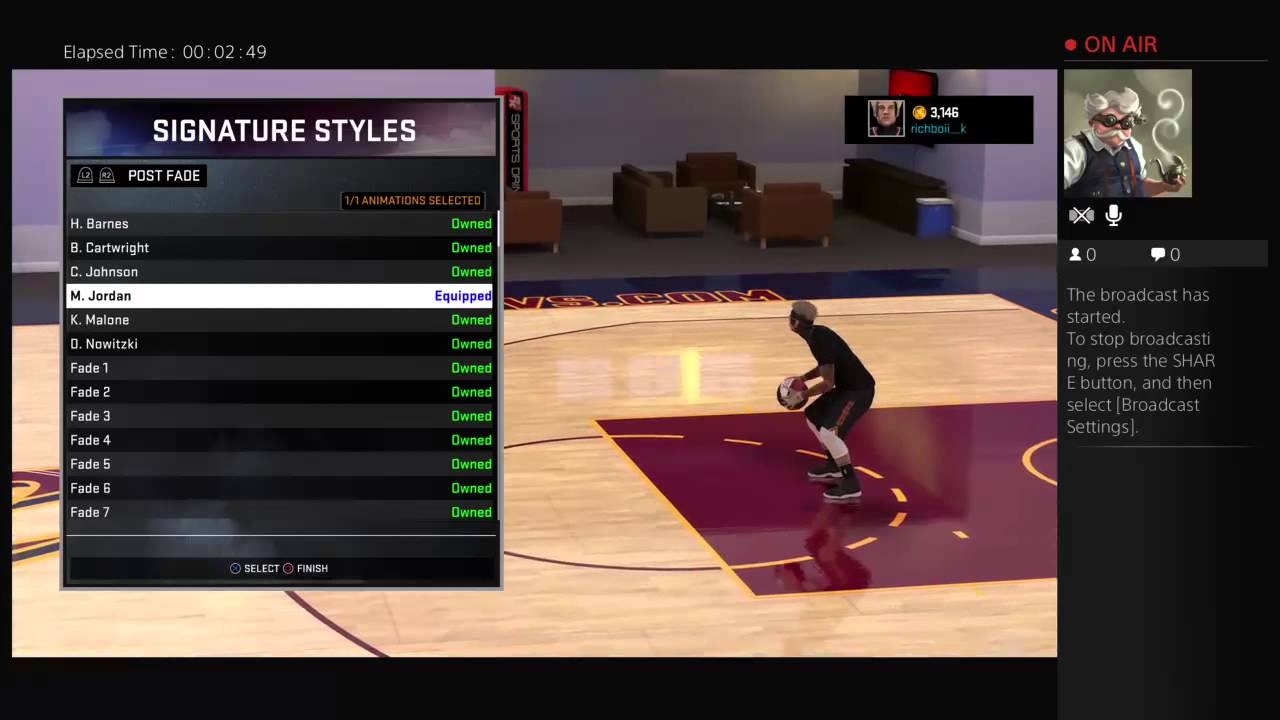This detailed caption has been cleaned up to offer a clear and descriptive overview of the screenshot from the video game:

---

In this screenshot from a basketball video game, likely being run on the BlueStacks emulator, a streamer named "Rich Boy," who has an avatar resembling a steampunk Colonel Sanders, is broadcasting live. The broadcast interface suggests that viewers can start and stop the stream by pressing the share button and adjusting broadcast settings.

The image captures a moment in the game where a black basketball player, dressed in black shorts and a black top with white gloves and a white headband, is positioned within the free-throw area of the court, marked by a red square. On the left side of the screen, there's a "Signature Styles" menu featuring various selectable basketball moves, including notable names like H. Barnes, B. Karth, C. Johnson, and K. Malone.

Michael Jordan's signature style is currently equipped, and the menu offers a variety of fade-away shots labeled one through eight. The menu indicates that "Rich Boy" possesses all listed signature styles, but has only activated Michael Jordan's moves.

The bottom part of the screen shows the PlayStation controller interface, with options to select (X) and finish (square), confirming that the game is being played with a PlayStation controller.

Overall, this detailed scene gives a comprehensive look at the game's signature style customization menu and the current status of the player's selected moves.